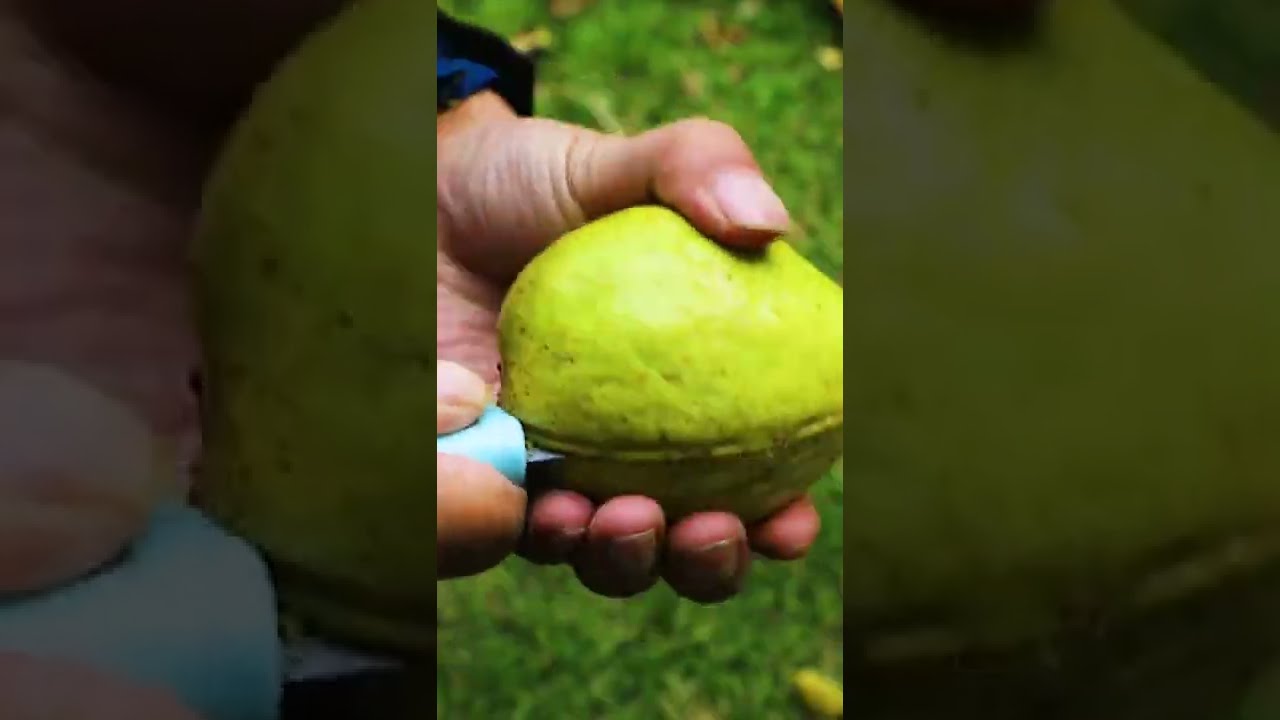In this close-up photograph set outdoors, a person with light skin is seen using their right hand to hold a blue-handled knife, which is inserted horizontally into a fruit held by their left hand. The fruit is green, shiny, and oblong, resembling the shape of an avocado but with the vivid color of a green apple. The central focus of the photograph captures the moment the knife penetrates the fruit, creating a clear horizontal cut. The background consists of blurred grass, contributing to the outdoor setting, and is overlaid by a digitally altered, enlarged, and darkened portion of the fruit, divided into two sections on the left and right sides of the image. This enlargement emphasizes the texture and color contrast of the green fruit, providing a striking backdrop to the central action of slicing.